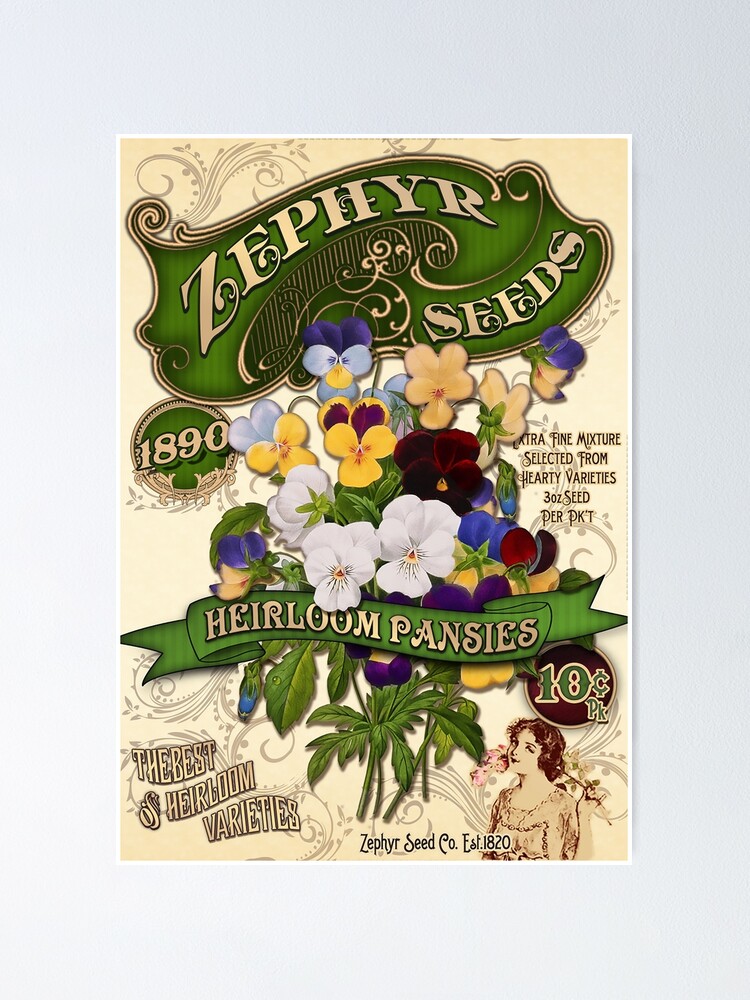This advertisement for Zephyr Seeds showcases a vintage-inspired design reminiscent of early 1900s aesthetics, featuring intricate curl and dot patterns and stylized banners. The image prominently displays "Zephyr Seeds" at the top on a green background, with "Heirloom Pansies" written across a central banner. The heirloom pansies in the illustration are vividly colored in purple, white, yellow, red, blue, and burgundy. Between the banners, there are decorative illustrations of the pansies and a vintage portrait of a woman suggesting a bygone era. Additional text on the left says "1890" in a green circle, and on the right, it says "Extra fine mixture selected from hardy varieties, three ounces of seeds per packet." At the bottom, another banner reads "The best of heirloom varieties, Zephyr Seed Co., established 1820." Finally, the price is marked as "Ten cents a pack," with the number ten highlighted in green on a purple circle.